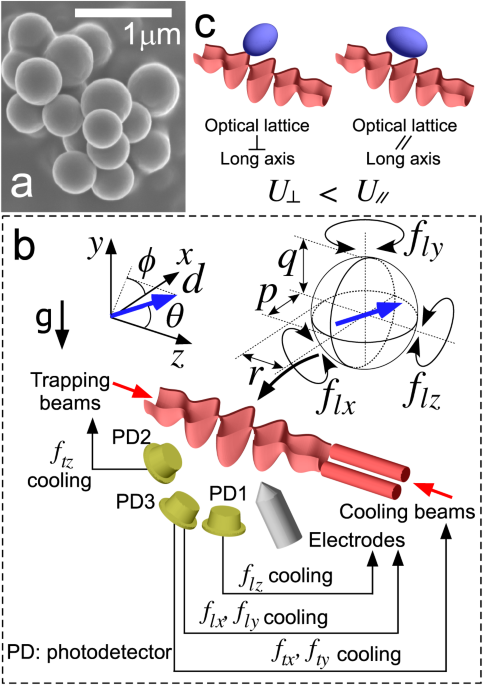This rectangular diagram is approximately 5 to 6 inches high and 4 inches wide, with a plain white background and no distinct border. It is divided into two main sections: a top third and a larger bottom section. 

In the top left section, labeled as "A," there's a small gray square filled with clusters of light gray bubbles, outlined in lighter gray and darker gray centers. In the lower left corner of this square, there is a lowercase "a" printed in white, and above the square, a white bar reads "1UM."

To the right of this, labeled as "C," are two side-by-side blue ovals with red ribbon-like bands underneath them. These ovals depict an "Optical Lattice Long Axis" view. The oval on the left has an upside-down "T" between the terms "Optical Lattice" and "Long Axis," while the right oval has two lines slanted diagonally upward to the right. Underneath these ovals, a formula is mentioned: "U with the upside-down T is less than U with the two diagonal lines."

The bottom portion, labeled "B," is more complex and detailed. It includes a dotted gray line outline in the upper left corner and various diagrams. One diagram shows an angle labeled with axes "Y," "X," and "Z." There's also a globe with arrows encircling it and additional letters like O, P, Q, and R. The "trapping beams" and "cooling beams" of the ribbons are also illustrated with lights going into them, indicated by arrows. Further down, it mentions "Electrodes" and "Cooling," with a specific note on "PD Photodetector" in the lower left corner. The section concludes with yellow button-like objects labeled "P1" and multiple "PD" labels (PD1, PD2, PD3).

This image appears to be a detailed scientific diagram, likely used as a visual aid for a presentation, showcasing various labeled components and complex interactions between them.